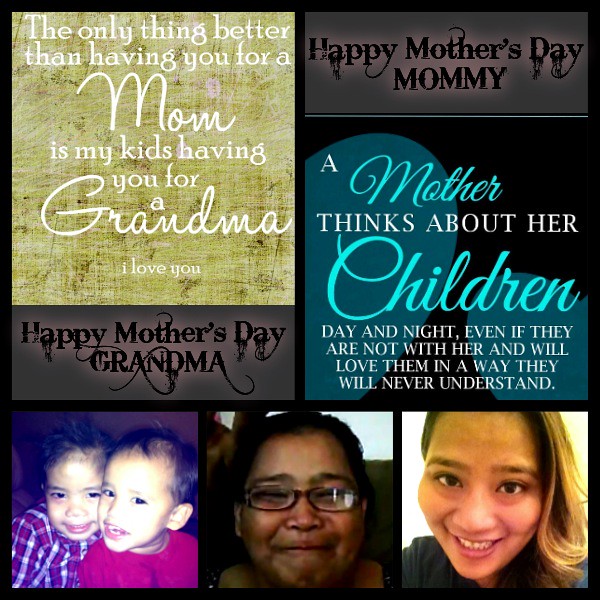This image is a detailed collage of seven scenes, forming a heartfelt Mother's Day tribute. In the upper left-hand corner, there's a quote in white cursive lettering on a greenish-white background that reads, "The only thing better than having you for a mom is my kids having you for a grandma. I love you." Just to the right of this, it says "Happy Mother's Day, Mommy" in bold font. Centered in the middle is another touching message: "A mother thinks about her children day and night, even if they are not with her and will love them in a way they will never understand."

On the lower portion of the image, three distinct photos capture precious family moments. To the left, there are two young children, likely around 4 to 6 years old, looking joyous. In the middle is the grandmother being honored; she has a warm smile and is wearing glasses. Finally, to the far right, there is a smiling woman who is the mother, expressing her love and appreciation in this Mother's Day card dedicated to her mom. The overall color palette includes shades of black, brown, white, tan, light blue, dark blue, gray, red, and purple, creating a visually appealing and emotionally resonant gift.